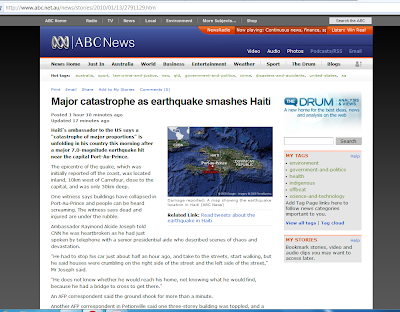This image showcases a desktop version of the ABC News website. 

At the very top of the page, the URL bar is visible, indicating the webpage being viewed. Directly below that is the website's main navigation bar on a gray background. The navigation options listed include: ABC Home, Profile, TV, News, Local, Environment, More Subjects, and a search box labeled "Search ABC."

Following this, there's a section with a blue background. On the right side of this section, there's an orange banner with the partially readable text "Now Playing Something." Within the blue background to the left, the white text spells out "ABC News, Video, Audio, Photos," and below these, blue hyperlinks for Podcasts, RSS, and possibly Gmail can be seen.

Another menu bar sits just beneath this, although the text is less clear. Some discernible options include Justin, Australia, World, Business, Entertainment, Weather, Sport, and Blogs, accompanied by a small menu.

The main feature of the image is centered below this series of menus: a prominent news story headline reads "Major Catastrophe as Earthquake Smashes Haiti." Beside the headline, there is an infographic showcasing the impact of the earthquake in Haiti. To the right, there's an additional menu with several hyperlinks leading to various topics, enhancing the navigability of the webpage.